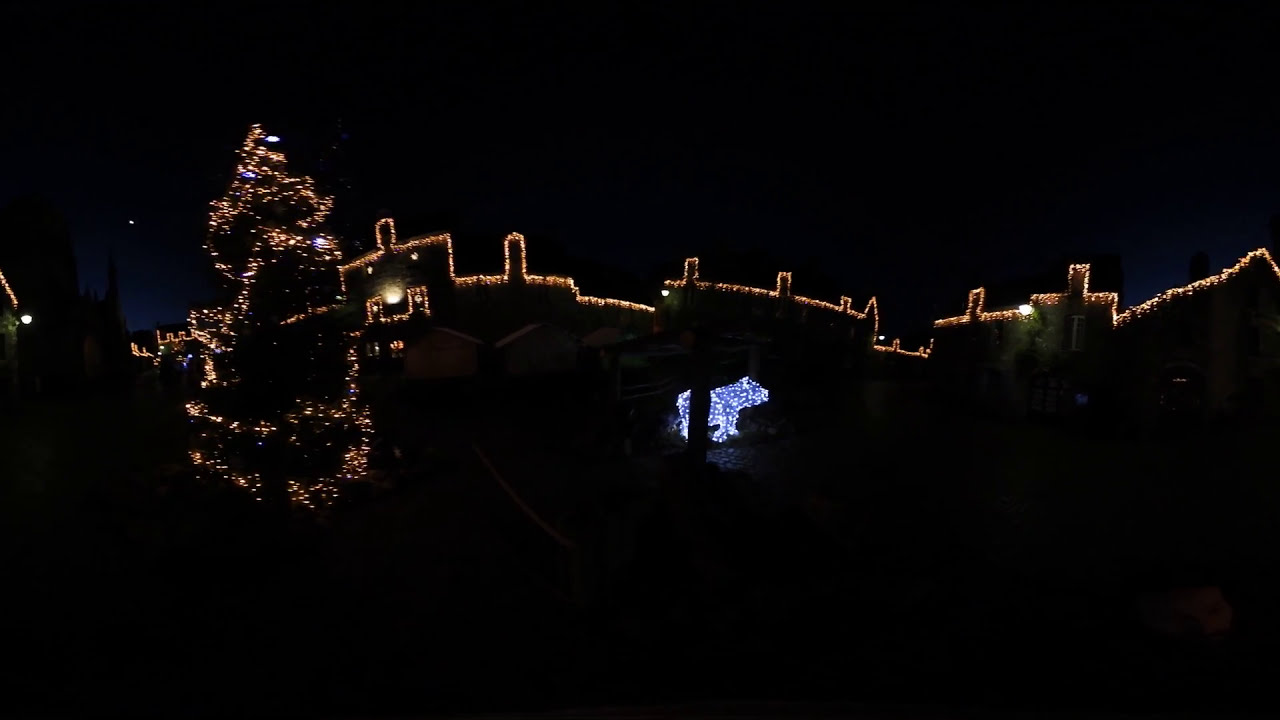The photograph captures a nighttime Christmas scene focusing on a house lavishly decorated with lights. The display, primarily featuring white and orange lights, traces along the roof's edge, moving in a complex pattern that includes slopes, steps, and straight segments. From the right side, the lights curve downwards and then ascend steeply, resembling a staircase. A striking bright white light marks a corner amidst these intricate light movements, before they continue upwards and leftwards, with occasional blank spots.

On the house's trim and over the doorways, the decorations extend leftward, culminating where a beautifully lit Christmas tree stands. The tree is adorned with yellow and green-blue lights, creating a spiraling effect typical of festive columns. 

At the center, the focus shifts to a figure resembling a polar bear, brilliantly illuminated in white lights and facing right. A black line intriguingly divides its lit body, adding a mysterious element to the scene. The background holds additional houses, dimly visible, punctuated by light borders along their roofs against the dusky, just-sunset sky. The overall ambiance is rich with holiday cheer, offering a delightful view of a festive home dressed for Christmas.